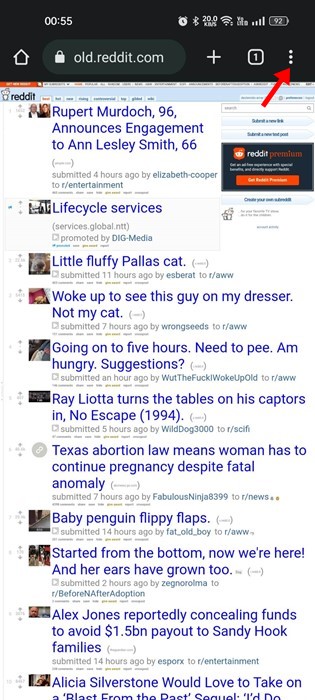A detailed screenshot of a smartphone displaying a website is captured. The phone shows a battery life of 92% and a strong network connection. The time on the device reads 00:55. In the browser’s search bar, the URL "old.reddit.com" is visible, accompanied by a plus sign on the right, a lock icon on the left, and a home icon. There are additional icons, including another plus sign, a square containing the number one, and a menu represented by three vertical dots. A red arrow points from the search bar to the three dots, indicating they are being highlighted.

The webpage displayed lists various articles. Featured articles include topics such as Rupert Murdoch, lifestyle services, a "little fluffy palace cat," someone waking up to see the sky with a dress that isn’t theirs, statements like "going on to five hours need to pee" and "am hungry suggestions," a mention of Ray Liotta turning the tables on his captors, a comment on Texas abortion law forcing a woman to continue a pregnancy despite fetal anomalies, and a whimsical mention of a "baby penguin flippy flaps." The list continues with more articles running down the page. 

The image itself is cut off, indicating that scrolling would be necessary to view the entire content. Additionally, at the top of the screen, there is a pop-up Reddit message notification.